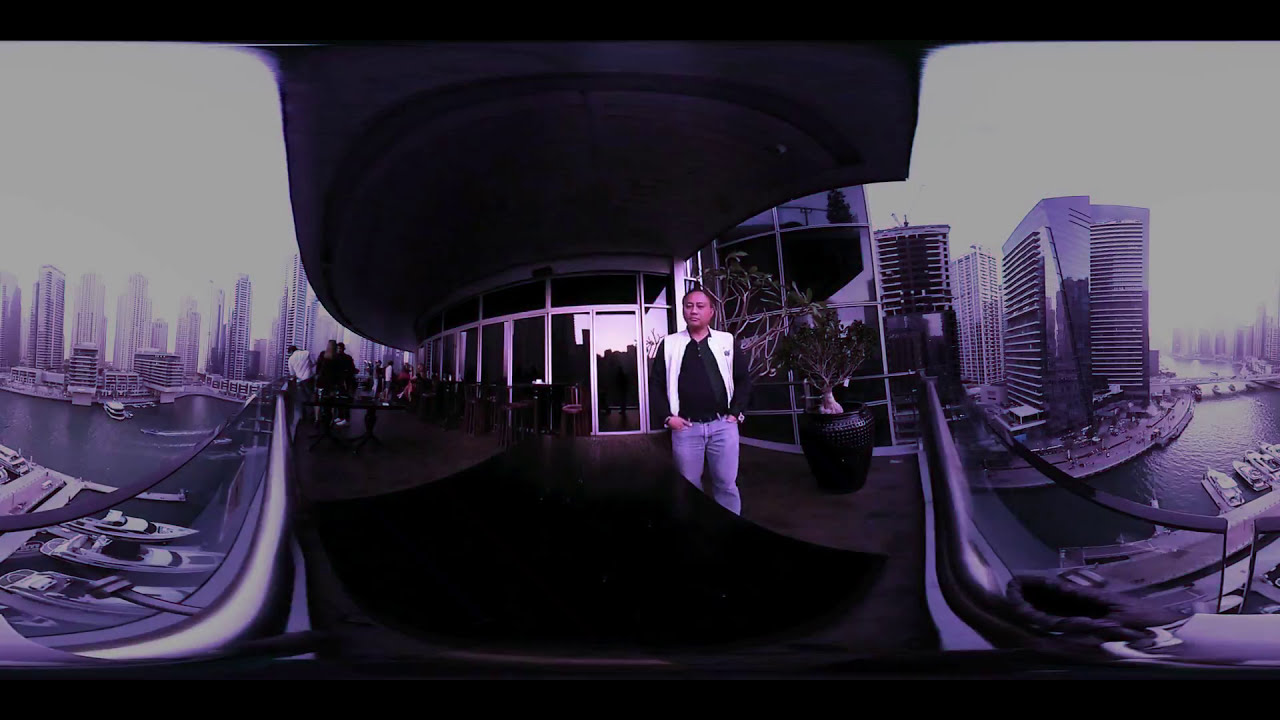The image captures a drab, overcast day from the perspective of an outdoor balcony or observation deck on a towering skyscraper in a sprawling city, which could resemble the skylines of Tokyo or Hong Kong. The deck is adorned with glass or plexiglass railings with silver accents, and tables and chairs where several groups of people are seen interacting. A notable feature is a large black pot holding a bonsai tree. Central to the composition is an Asian man standing on the balcony, hands in his pockets, dressed in blue jeans, a black button-up shirt with long sleeves, and a white vest. Behind him, a wall of horizontal and vertical windows can be seen. Below the balcony, there's a vast body of water dotted with various boats, including white speedboats and larger yachts docked along the side. The fisheye lens effect slightly distorts the image, giving it a unique curvature. The scene is further framed by an array of distant skyscrapers stretching towards the grey sky.